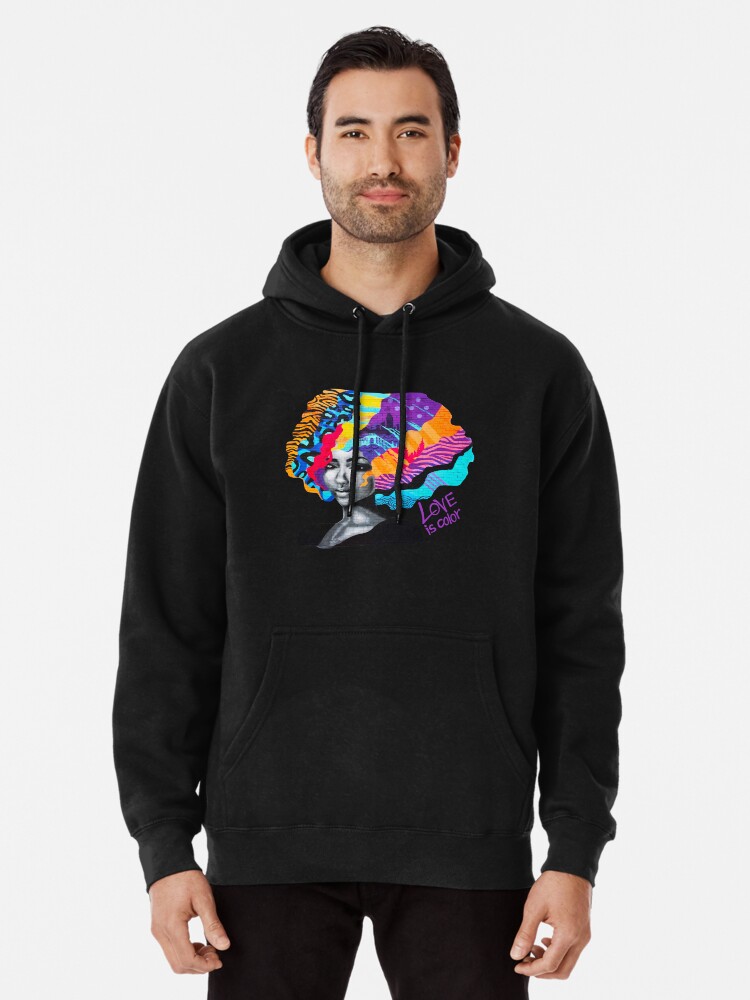The image features a man standing against a light blue background, illuminated well enough to see fine details. He has a lighter skin tone, short black hair, thick black eyebrows, and dark eyes. His face is adorned with stubble that covers his lower face but does not form a full beard or mustache. He is wearing a black hoodie, with the hood down and two strings hanging from the neckline. The hoodie is in good condition and features a colorful design on the front. The design depicts a woman's face with hair made up of a collage of colors, including blue, yellow, pink, purple, and orange. The image also includes the phrase "Love is Color" at the bottom right of the colorful hair. The man is also wearing black pants that resemble sweatpants. He stands facing the camera, with his arms relaxed at his sides, extending to the upper thigh area. His posture is straightforward, as if posing to model the outfit.